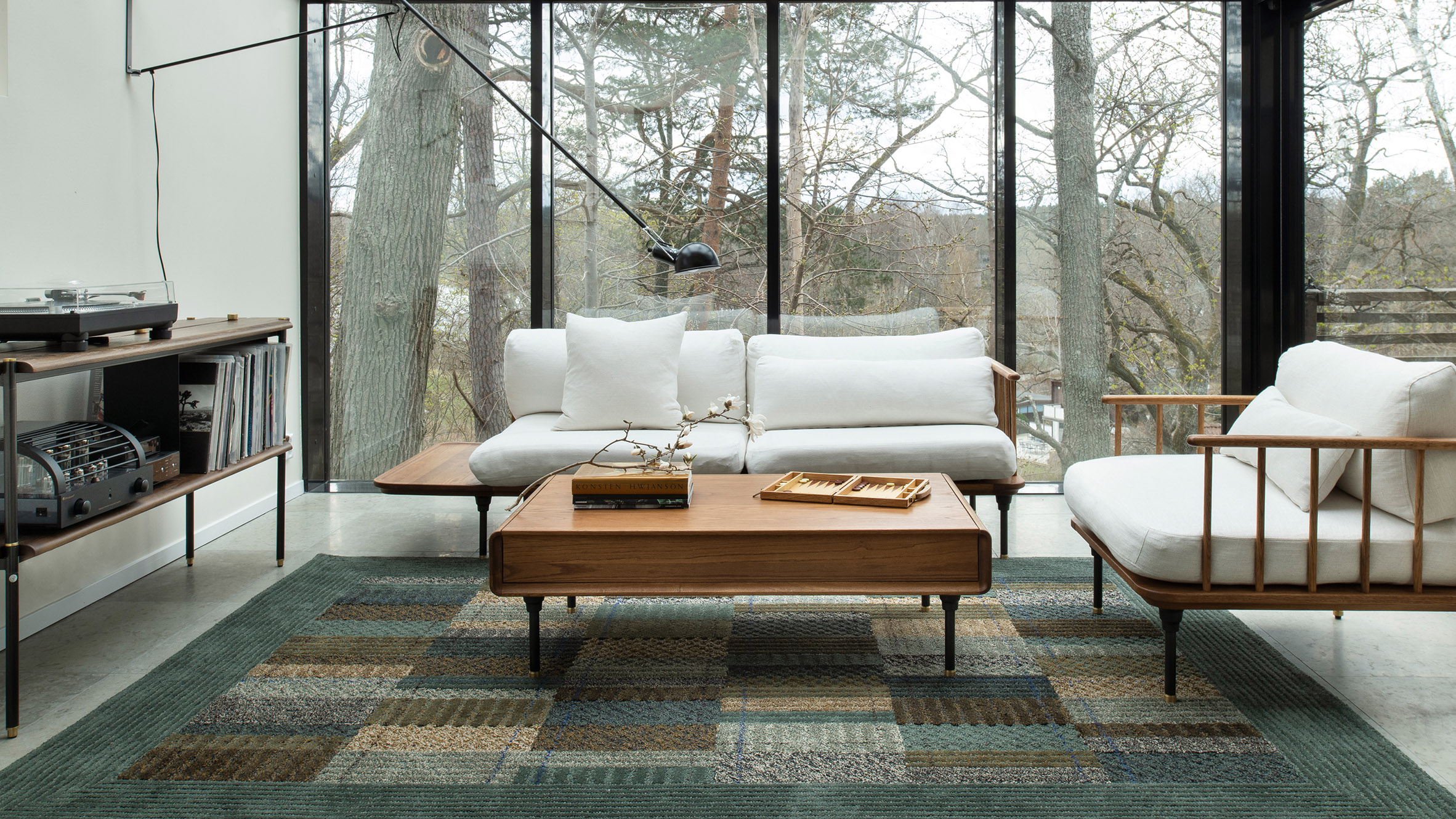The photo captures a cozy living room set in a modern home nestled in a forest of both evergreen and deciduous trees, evident through the large floor-to-ceiling windows on at least two sides of the walls. The natural light streaming in, despite an overcast sky, brightens the room with a cool ambiance. The focal point of the space includes two short, white-cushioned couches arranged around a wooden coffee table. The table itself is adorned with an elegant twig with blossoms placed over two books, alongside a small wooden tray or box. A dark yet colorful rug with a green border and a quilt-like pattern of varied hues including dark grays, greens, browns, and splashes of black and white covers the floor.

To the left of the seating area, a wooden shelf stands against a white wall, housing a turntable, with records or books underneath it, and an intricate machine with black knobs, and another small wooden box. An eye-catching feature is the large black desk lamp, which seems to extend from the wall or ceiling to illuminate the coffee table area. The minimalist yet sophisticated decor harmonizes well with the serene outdoor landscape visible through the expansive windows, further enhancing the sense of tranquility and seclusion on this slightly gray, yet luminous day.